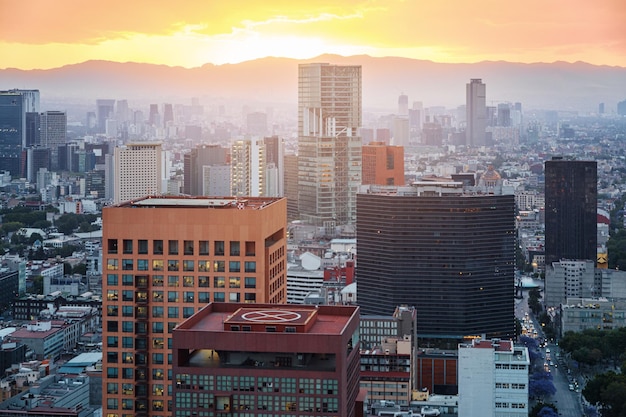The photograph captures a captivating city skyline at either sunset or sunrise, as the sky is bathed in a dreamy peach and golden hue. The scene is slightly hazy, enhancing the ethereal atmosphere of the image. Dominating the landscape are numerous skyscrapers and buildings constructed from glass, brick, stone, and various shades of gray, beige, and red. Prominent structures include a large red building with a helipad marked by a white circle and cross, a black skyscraper, and another large, gray skyscraper. Nestled among these are smaller white, gray, and red structures. In the background, a faint silhouette of a mountain range adds to the grandeur of the scene, blending seamlessly with the horizon where the sun casts its orange and yellow glow across the entire sky. The bottom part of the image reveals a bustling street far below, dotted with tiny cars, completing this busy and vibrant urban snapshot.